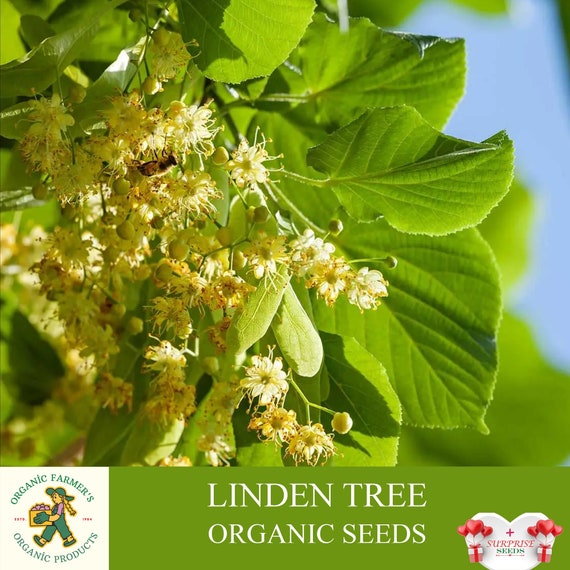The image is a digitally presented package cover for a product, likely Linden Tree Organic Seeds. Dominating the cover is a vibrant, close-up photograph of a linden tree branch adorned with detailed green leaves, their veins clearly visible. Among the leaves are white and yellow seeds sprouting in various areas, some of which are accompanied by blooming flowers and even a bee. The background fades into a blur, suggesting a sunny, clear day with a visible blue sky towards the right side. Underneath the main image, a green band displays the text "Linden Tree Organic Seeds" in white. On the lower left, a white square features the logo of Organic Farmers, showcasing a girl with long blonde pigtails, wearing green overalls, a big hat, and gloves, carrying a box of vegetables. Overall, the package design blends rich botanical details with clear product branding.